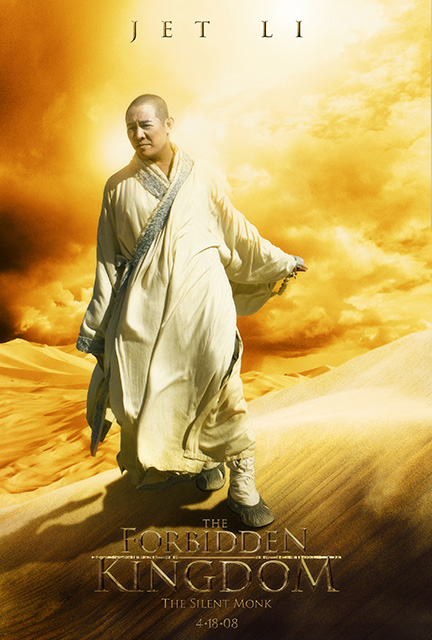This color photograph is a detailed movie poster for "The Forbidden Kingdom, The Silent Monk," starring Jet Li. The release date, prominently displayed at the bottom, is April 18, 2008. In the center of the image, Jet Li stands on what appears to be yellow and orange sand dunes, beneath a sky of similar hues with scattered clouds. He wears flowing white monk robes, paired with hospital shoe-like slippers and fluffy socks, with one foot bare. Jet Li’s head is shaved close to the skin, and he gazes thoughtfully into the distance. The text above him reads "Jet Li," emphasizing his starring role, while the title of the movie and its release date are centered at the bottom. The overall scene conveys a contemplative yet poised atmosphere, highlighting Jet Li's ready stance amidst the serene yet dramatic landscape.